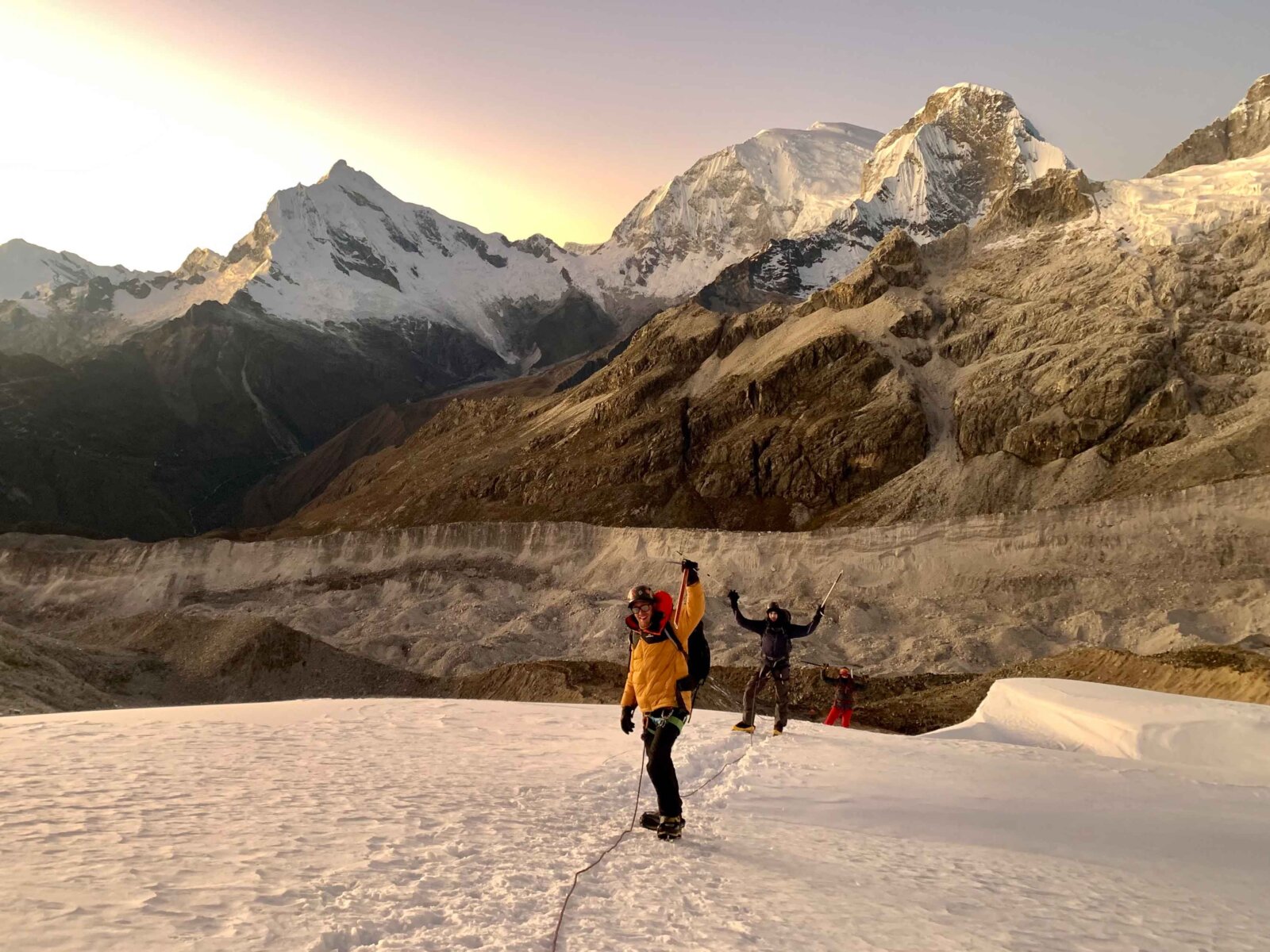In this landscape photograph, a group of three people are captured mid-hike on a snowy glacier, surrounded by a majestic mountain range. The foreground features a flat expanse of snow, stark white and stretching across the lower third of the image. The central figure, facing the viewer, wears black pants and an orange jacket, raising his left arm which holds an ice pickaxe. He is secured with a rope tied to his waist that extends across the snow. Behind him, another hiker, dressed entirely in black, also raises an ice pickaxe. Further back, a third person, clad in a brown jacket and red pants, raises both arms, seemingly gesturing. All three are equipped with short hiking poles and are tethered together by a safety rope. 

The background reveals a dramatic mountainscape; jagged, snow-covered peaks rise toward the sky. The closest peak, dark with only a dusting of snow at its tip, contrasts with the more distant mountains, which are heavily layered with snow. Approximately 20% of the image at the top is occupied by a sky with a partial sunny spot on the left, casting a subtle rainbow-like line down into the mountains. The photograph’s realistic style captures both the climbers’ vibrant attire and the breathtaking natural scenery in vivid detail.